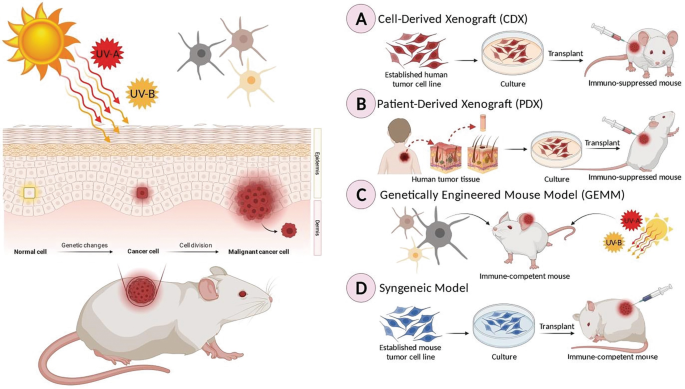The diagram is divided into two primary sections. On the left side, a vibrant yellow and orange sun emits rays depicted in shades of yellow and red. These rays are directed toward a detailed, close-up illustration of human skin layers, highlighting the effects of ultraviolet radiation. Labels next to the sun indicate "UVA" on a red background and "UVB" on a yellow background. Within the skin illustration, there's a conspicuous large red spot marked as a "malignant cancer cell." Below this, an image of a white mouse with a pink tail also has a similar red spot on its back, suggesting a shared pathology.

The right side of the diagram contains four subsections labeled A, B, C, and D, each detailing different methods related to cancer research using mouse models. Section A, "Cell-Derived Xenograft," describes the process starting from an "established human tumor cell line," moving to culture, and then to transplanting this into an "immunosuppressed mouse," illustrated with an image of the mouse. Section B, "Patient-Derived Xenograft (PDX)," follows a similar path but starts from "human tumor tissue." Section C, "Genetically Engineered Mouse Model (GEMM)," involves an "immune-competent mouse." Lastly, Section D, "Syngeneic Model," begins with an "established mouse tumor cell line," which is cultured and then transplanted into an "immune-competent mouse."

In summary, the diagram provides a comprehensive overview of the interaction between UV radiation and skin cancer development, alongside the various mouse models used in cancer research to study tumor growth and response.